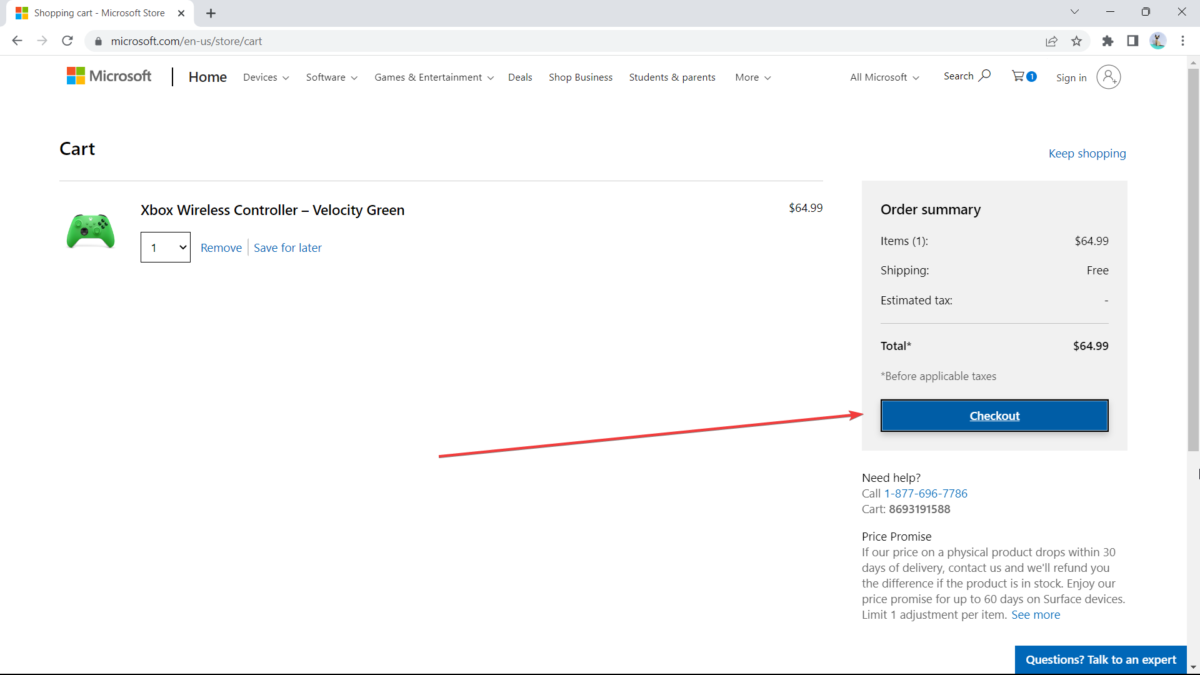This is a detailed screenshot of a Chrome browser window with a single open tab displaying the Microsoft Store's shopping cart. The address bar is visible at the top of the window, and a user profile picture featuring a cat is located at the far right. 

The main content of the webpage shows a shopping cart containing an "Xbox Wireless Controller - Velocity Green" with a quantity set to one. Next to the quantity box are options to "Remove" or "Save for later." A picture of the controller is positioned to the left of the item title.

On the far right of the webpage, there is an "Order Summary" section highlighted by a prominent red arrow pointing towards the blue "Checkout" button. The total cost for the item is $64.99, and shipping is listed as free. Above the order summary box, there is a "Keep shopping" link. 

Below the order summary, a "Need Help?" section provides a phone number for customer support, a cart number, and a "Price Promise" guarantee. At the bottom right corner, there is a blue tab labeled "Talk to an expert," which offers users the option to ask questions and receive additional assistance.